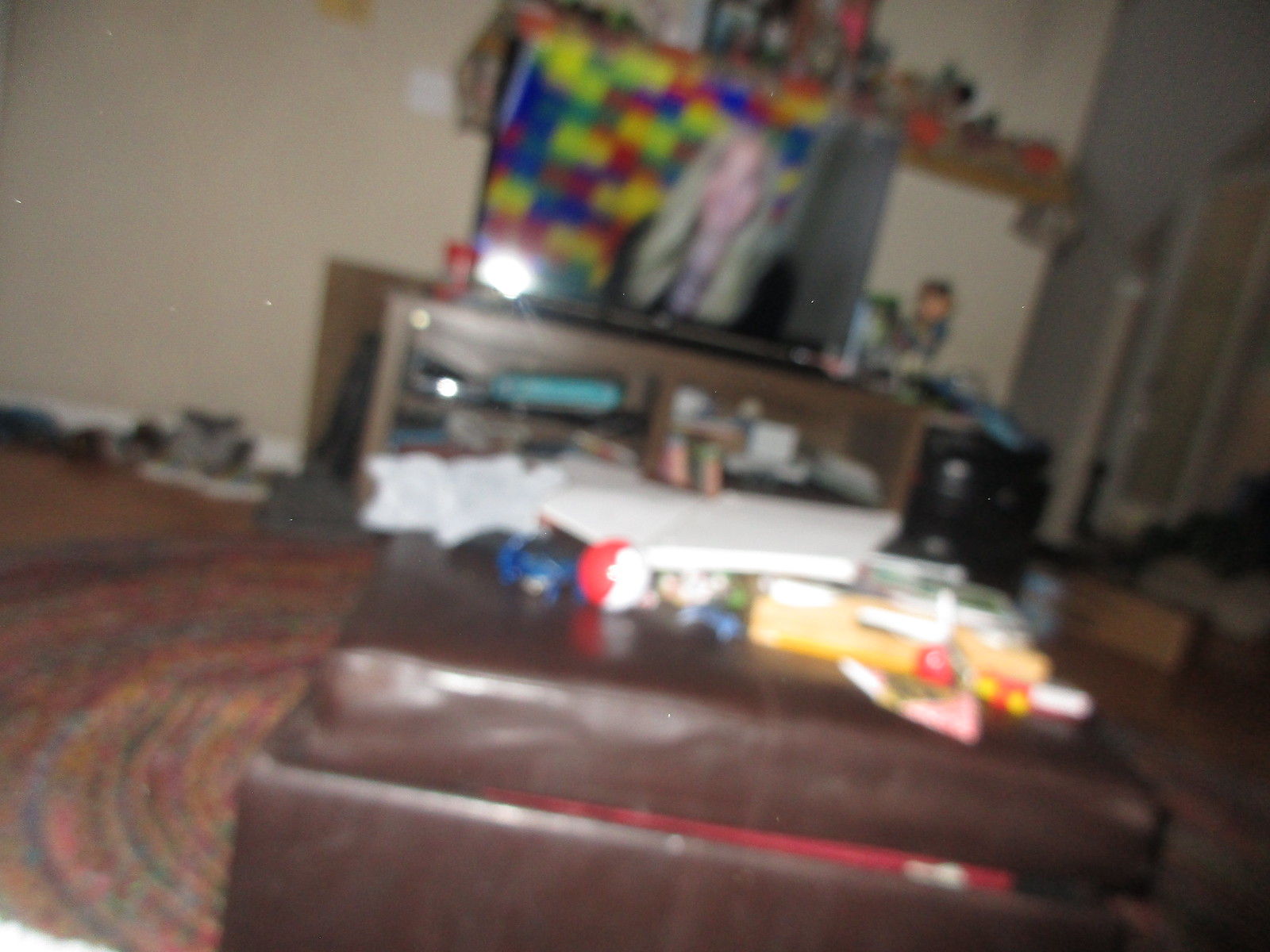The slightly out-of-focus image captures an indoor living room scene. Dominating the floor is a circular, multicolored braided carpet with predominant hues of red and blue. At the forefront and center of the image is a green storage ottoman, its lid slightly ajar to the right, revealing a glimpse of red fabric inside. Piled on top of the ottoman is a stack of papers and miscellaneous items, including a manila envelope and possibly some flowers with red petals and yellow centers. There is also a roll of paper, half red and half white, amidst the clutter.

Against the far wall stands a credenza with several shelves displaying blue objects and books, supporting a flat-screen TV. Above the TV, a brown wall shelf holds various black, white, and red items. To the right of this setup, a black filing cabinet is visible, also topped with a variety of items. The wall to the left of the TV turns and extends downwards, featuring beige-white baseboards. Near the baseboard, there are additional items scattered on what appears to be a wooden floor underneath the colorful carpet.